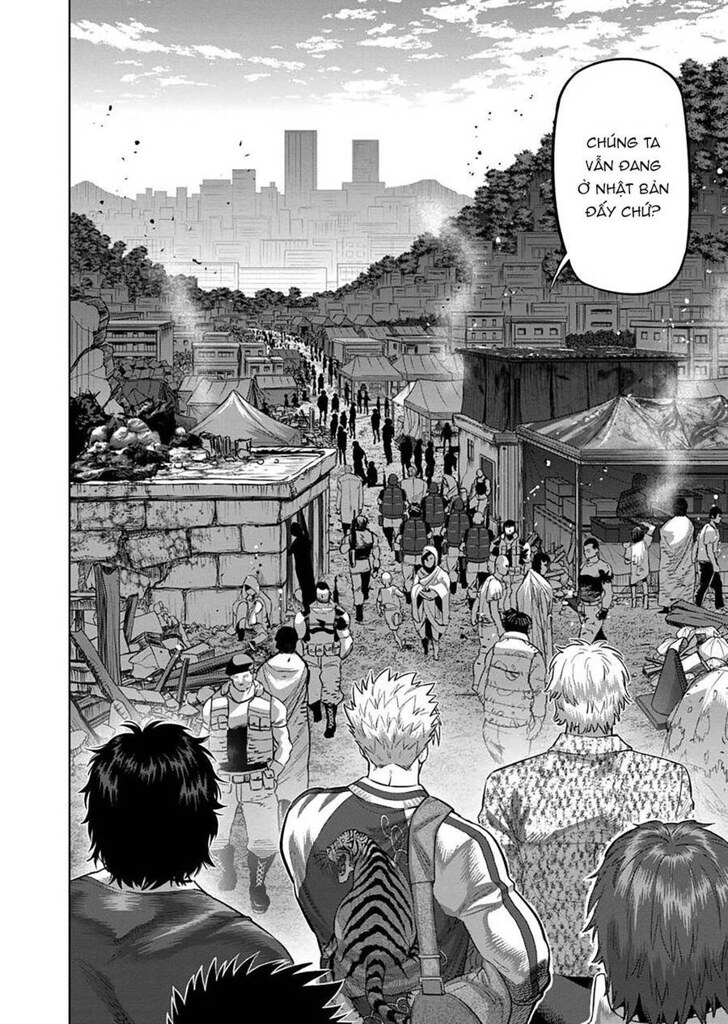The image appears to be a scan of a black-and-white manga or graphic novel page. At the bottom of the panel, we see a group of characters, possibly the protagonists, walking into a village that resembles a modern-day slum. This area, filled with tents and smoky surroundings, indicates a war-torn, economically struggling community. Among the characters, one stands out wearing a jacket with a tiger emblem on the back and carrying a bag. The group includes individuals with varying hair colors: light brown, blondish, and dark black.

In the scene, the streets are populated not only by civilians but also by armed military officers, suggesting a high-security presence or possible evacuation efforts. As the characters advance further into the village, the art transitions to less detailed silhouettes, emphasizing the depth and vastness of the setting. A food stand can be seen, and some characters appear to stop there, adding a touch of normalcy amidst the chaos.

In the upper right corner of the panel, there is a speech bubble containing text in an unfamiliar language. The overall grayscale palette of the illustration further enhances the somber and gritty atmosphere of the scene.